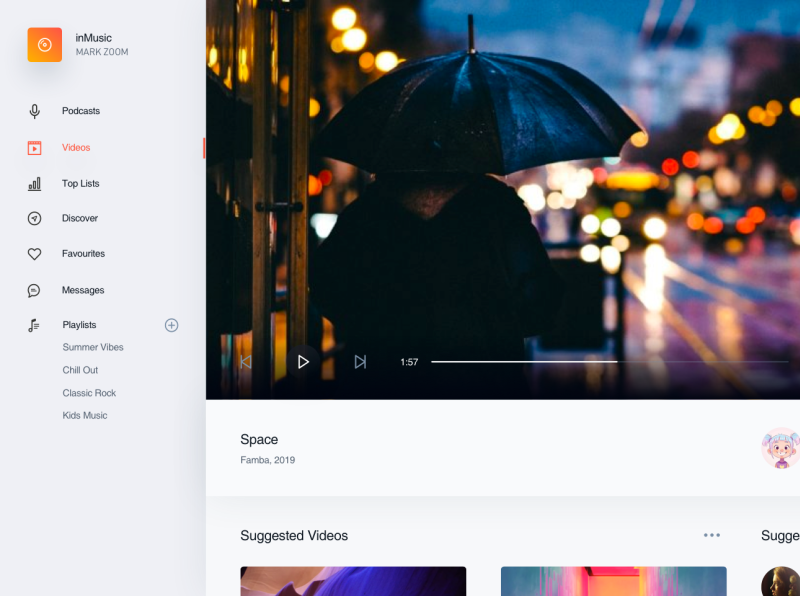This image captures a detailed layout of a multimedia website interface with varied sections and elements. From the left margin, about two inches inward and extending down to the bottom, the background is a light gray color. Situated an inch below the top left corner, there is a prominent orange square, containing a white-bordered orange circle with a white center. To the right of the circle, in black text, it reads "In Music," and directly below in a slightly lighter black font, it says "Mark Zoom." 

Moving downward, there is a voice icon accompanied by the label "podcast" in black. Adjacent to this is a video icon labeled "videos" in red. Further below, there are icons each with corresponding labels, including "top list," "discover," "heart," "favorites," "messages," and "playlists." Under the "playlists" label, in a lighter color, is a list of playlist names: "Summer Vibes," "Chill Out," "Classic Rock," and "Kids Music."

To the right of these lists, an image spans approximately two-thirds of the page height. It depicts a nighttime city street scene with rain, where a person, dressed in black, holds a black umbrella. Car lights approach from the background, and buildings can be seen to the left. Positioned over this image are playback controls; a play button on the left, with rewind and fast-forward buttons on either side. To the right, a white progress bar extends halfway across the page, marked "1:57" at the left end. Below this bar is an inch of white space, containing the text "space" on the left and "Famba 2019" beneath it.

On the far right side is the icon of a drawing depicting a little girl with blue hair, wearing a pink shirt, and smiling. This is bordered by a light gray margin that extends approximately two inches from the top. At the bottom left of this section, the text in black reads "suggested videos," switching to "S-U-G-G-E" to the right, followed by ellipses. Below this, the top edges of two more pictures are visible from left to right, alongside about half of a profile picture of a person gazing left, set against a black background.